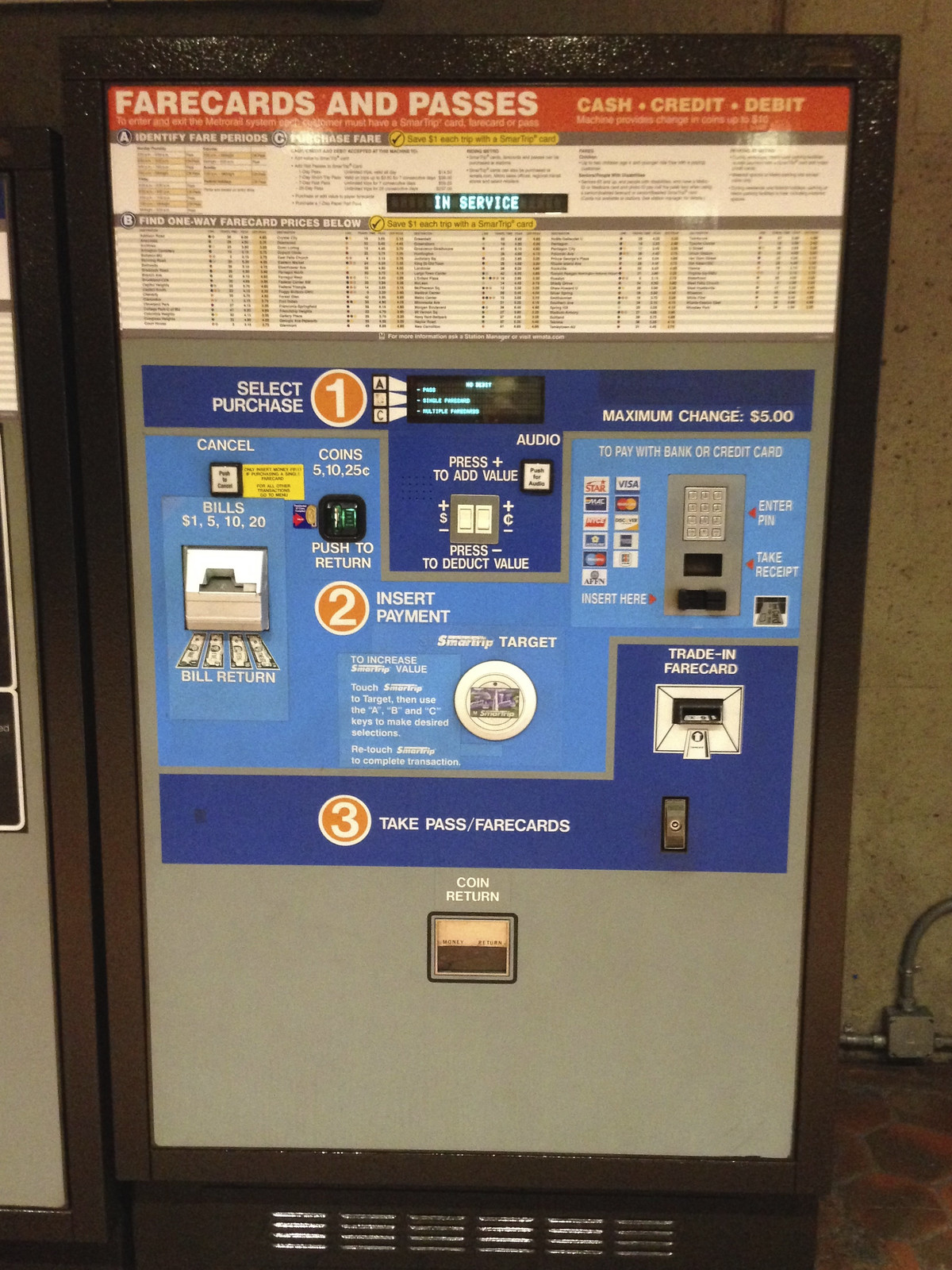The photograph features a centrally positioned, silver-colored fare card and pass vending machine at a metro or train station. This automated machine is designed to sell fare cards and passes, and it prominently displays instructive text in red and white, with visual backgrounds in blue to aid users. At the top of the machine, a label reads "Fare Cards and Passes," indicating that it accepts cash, credit, and debit payments. The machine's interface includes multiple buttons, a pin pad, and dedicated slots for coin and bill insertion, guiding users through a numbered step-by-step process to purchase fare cards. Steps involve identifying fare periods, selecting one-way fare card prices, inserting payment, and finally taking the printed pass or fare card. There is also a lit-up panel in blue letters confirming the machine is "In Service." Instructions and visual aids mounted above various sections facilitate user interaction, and there's a coin return slot and a designated area for retrieving the purchased fare cards or passes at the bottom. The maximum change given is $5, ensuring convenience for users handling cash transactions.